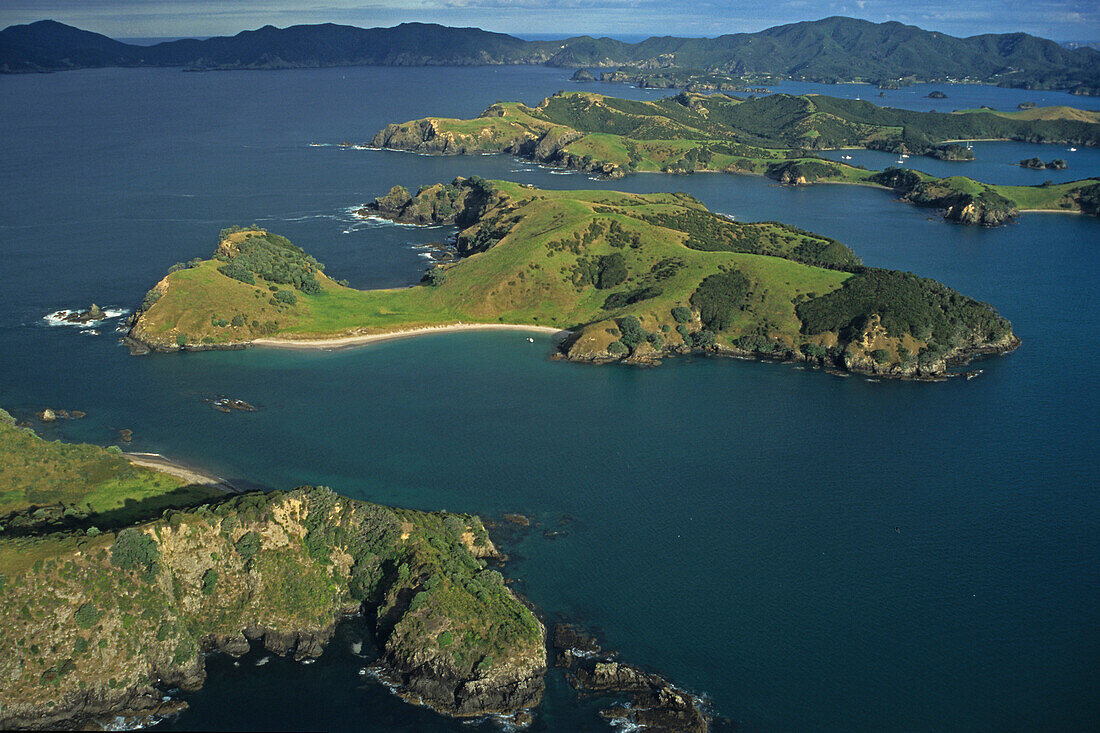This aerial photo showcases a serene cluster of non-symmetrically shaped islands surrounded by a vast expanse of calm, dark blue water. The scene is set on a sunny, clear day, enhancing the vibrant colors and details. In the foreground, there are three prominent islands, predominantly covered in grassy patches varying from light to dark green, interspersed with larger, darker green bushes and rocky outcroppings along their edges. Scattered clusters of rocks can be seen floating around the islands, enhancing their rugged charm. The bottom left corner of the image features a portion of the water, indicating the close proximity of these islands to one another. In the middle ground, between the islands, calm waters harbor a few small boats, and one island even has a small bay serving as an anchorage. The backdrop of this picturesque setting is a hilly, elongated strip of land stretching from the left to the right edge of the photo. This landmass transitions into a distant, undulating mountain range, emphasizing the area's tranquil and expansive watery landscape, with additional water visible beyond the hills.